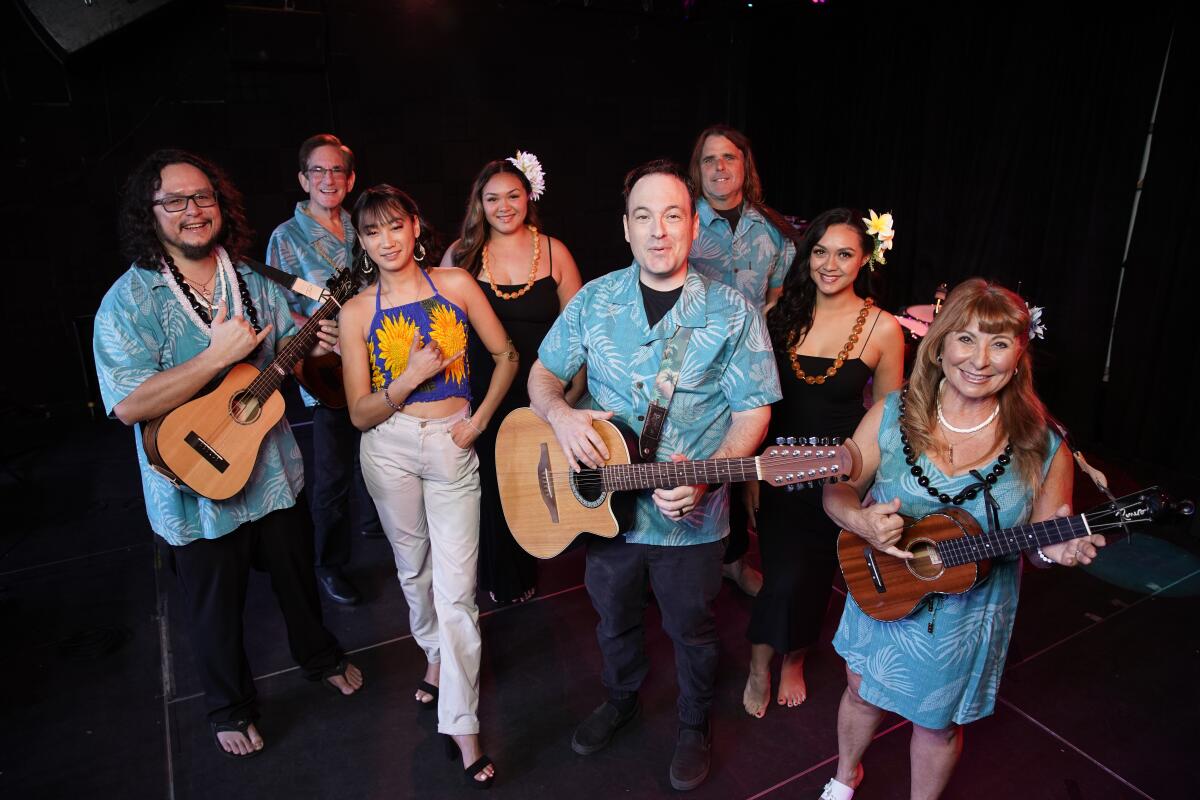The image depicts a vibrant mixed-age group consisting of eight people, four men and four women, posing happily in what appears to be a recording studio with black floors and walls. The men are uniformly dressed in light blue Hawaiian shirts adorned with white floral designs, paired with black jeans. Three of them hold guitars. The women display varied yet coordinated outfits: one mirrors the men's Hawaiian pattern in a dress form; another sports a black dress accented with brown or orange beads and a white flower in her hair; a third wears white pants, black high-heeled shoes, and a blue shirt decorated with yellow flower pieces; another also in a black dress, adorned similarly with a white flower and orange beads. The group, appearing ethnically diverse, with three Asian women, one Caucasian woman, three Caucasian men, and one Asian man, smiles warmly at the camera, suggesting a moment of celebration, perhaps after a performance or in anticipation of one.